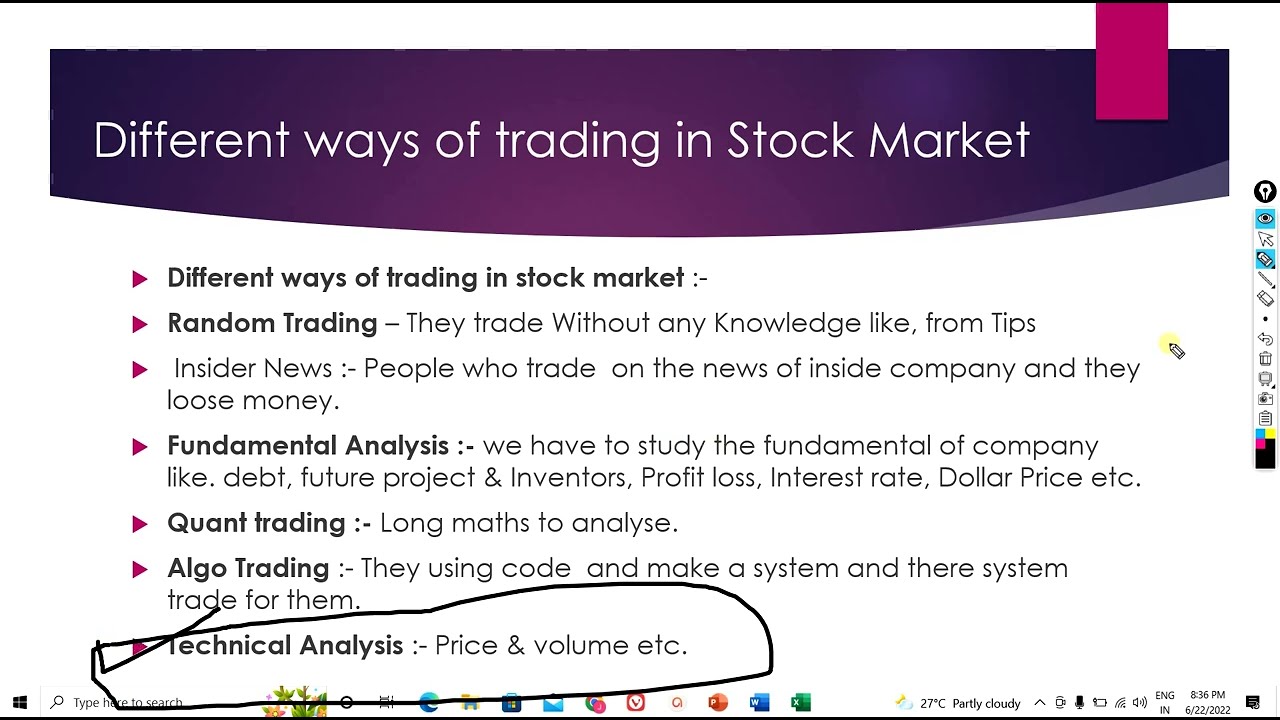This image is a detailed screenshot of a PowerPoint slide, likely part of a finance class presentation or notes taken by a student on different methods of trading in the stock market. The slide features a white background with a purple stripe at the top, containing the title in white text: "Different Ways of Trading in Stock Market." Below the title, several bullet points listed with pink triangle markers delineate the various trading methods:

1. **Random Trading**: Describing traders who act on tips or insider news without proper knowledge, often resulting in financial losses.
2. **Fundamental Analysis**: Emphasizes the need to study company fundamentals such as debt, future projects, investor information, profit and loss, interest rates, and dollar prices.
3. **Quant Trading**: Involves complex mathematical analysis to inform trading decisions.
4. **Algo Trading**: Utilizes coding to create automated trading systems that execute trades based on programmed strategies.
5. **Technical Analysis**: Focuses on analyzing price and volume data.

The slide also features a crude black circle drawn around "Technical Analysis" with a check mark beside it, indicating special emphasis or relevance. Additionally, the desktop screenshot reveals a typical computer interface bar at the bottom, showing elements like the "Type to search" box, Internet Explorer logo, weather information, and the current time.